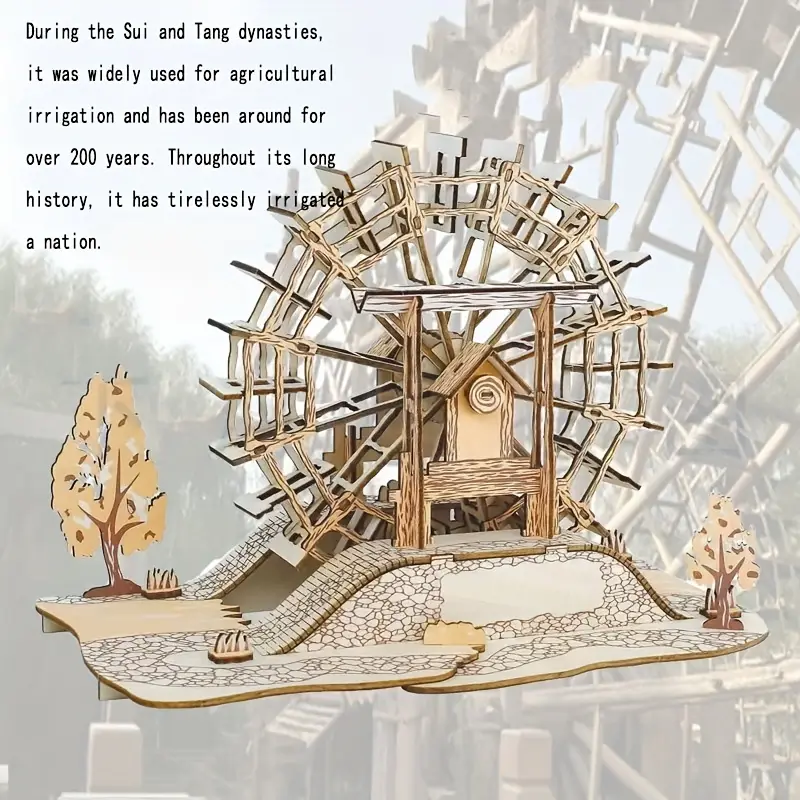The image depicts a detailed illustration of an agricultural irrigation system, specifically a wooden water wheel, prominently positioned at the center. The water wheel, rendered in light brown wood, stands amidst a backdrop that blends both realistic and illustrative elements. The background features a somewhat blurred replication of a real-life mill and nature scene, including another water wheel visible towards the right. Flanking the central water wheel are two trees, one on each side, with stone pathways surrounding the entire setup and leading up to a slight elevation, possibly representing a bridge or platform area. The top left corner of the image contains black text stating, "During the Sui and Tang dynasties it was widely used for agricultural irrigation and has been around for over 200 years. Throughout its long history, it has tirelessly irrigated a nation." This intricate depiction highlights the historical significance and enduring utility of the water wheel in agricultural practices during the Sui and Tang dynasties.